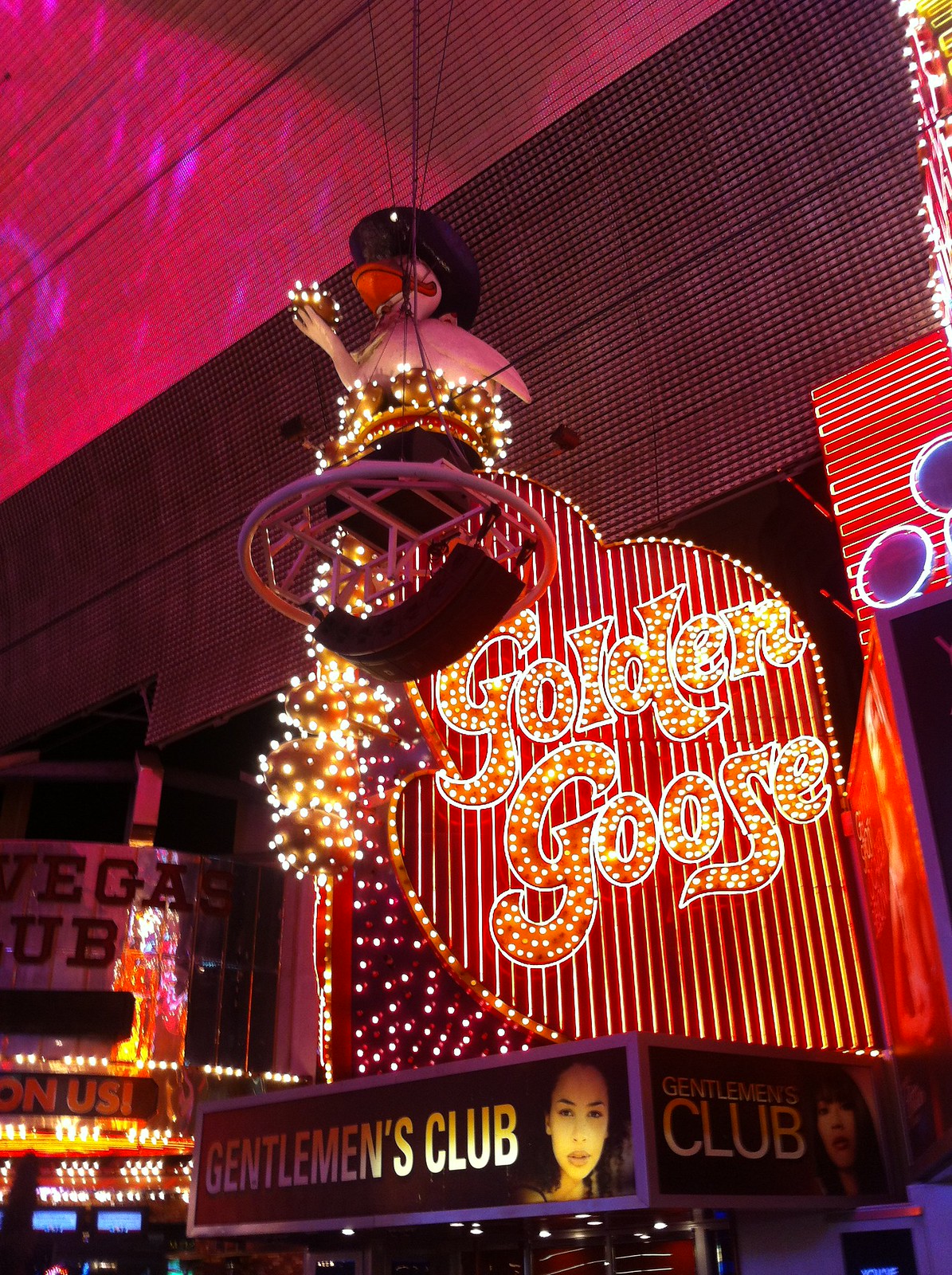The photograph depicts the bustling exterior of a business establishment, likely set in Las Vegas, known for its vivid and extravagant lighting. The focal point is a grand, illuminated sign emblazoned with the words "Golden Goose," glowing in an array of gold and yellow lights against a red backdrop. Above this vibrant text, a statue of a goose adorned in a cowboy hat, wrapped in festive Christmas lights, draws attention. Directly below the "Golden Goose" sign, a black marquee with golden lettering states "Gentleman's Club" and features the faces of attractive young women, who appear to be Asian. Additional decorations include clusters of purple and blue lighting that cast a colorful ambiance over the scene, while adjacent structures, partially visible, display fragmented signage including the recognizable word "Vegas." The setting appears to be outdoors, richly detailed and illuminated like a classic Las Vegas sidewalk, though partially covered by what seems to be a tile roof.